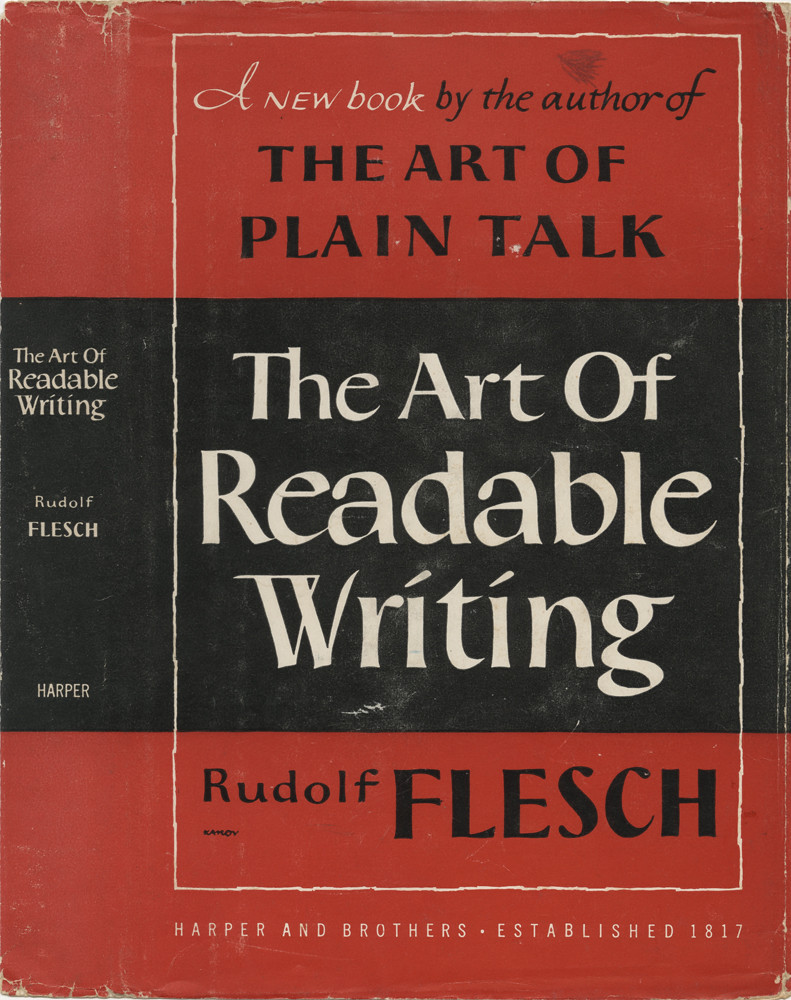This image showcases the front cover of an older book. The cover design is divided into three horizontal sections: the top and bottom are a dark red color, while the middle section has a black background. A white pinstripe rectangle frames the text in the central portion of the cover.

At the top, within the red section, white text reads "A New Book." Directly beneath it, in black text, it states, "By the Author of The Art of Plain Talk." The central area, with its black background, features the book's title, "The Art of Readable Writing," prominently displayed in large white letters. Below the title, still within the black section, the author's name, Rudolf Flesch, is printed in smaller black letters.

At the very bottom, also in white text, "Harper and Brothers, Established 1817," is displayed, indicating the publisher and its founding year. The book's spine echoes the cover's design, repeating the title "The Art of Readable Writing" in white text, along with the author's name, Rudolf Flesch, and the publisher, Harper.

The cover shows signs of age, with small white scuff marks visible on the black section, adding to its vintage appearance.